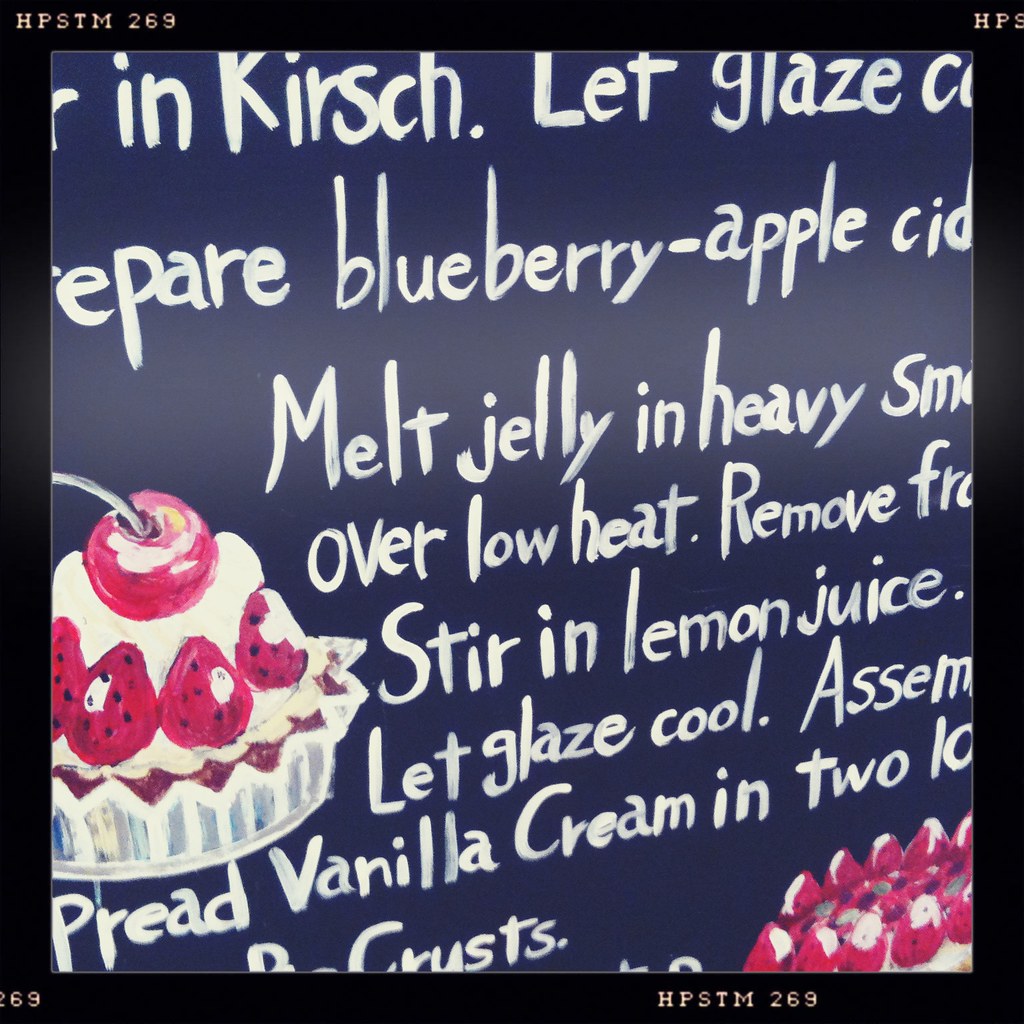A color photograph captures a charming, handwritten chalkboard recipe for a delectable dessert. The sign features a vibrant mix of illustrations and scripted text on a black background, framed by a black border adorned with small, light-colored text reading "HP STM 269." The recipe is partially legible: it begins with instructions to "encirche, let glaze, prepare blueberry-apple... melt jelly in heavy... over low heat. Remove. Stir in lemon juice. Let glaze cool. Assemble. Spread vanilla cream..." Unfortunately, some text at the edges of the image is cut off due to close zoom.

In the bottom right corner, the board showcases delightful chalk illustrations, using colored chalks for vibrancy. Depicted are circular tart dishes filled with cream, strawberries, and cherries, bringing the recipe to life visually. Amid this culinary artwork, the experience is reminiscent of an artisanal ice cream parlor or dessert café, blending rustic charm with mouth-watering imagery.